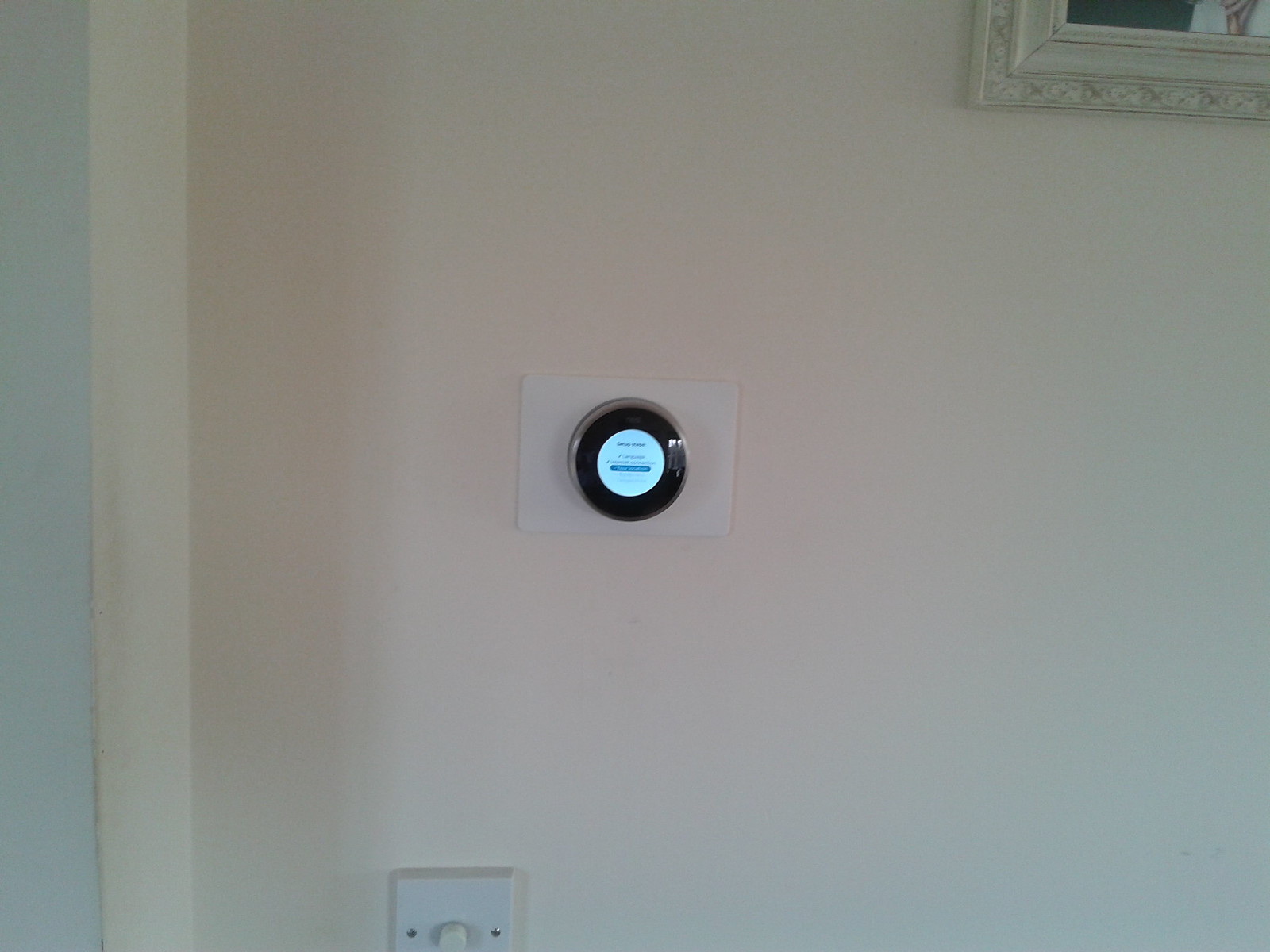This photograph captures a modern, technologically advanced interior setup. The central focus of the image is a sleek, circular smart thermostat mounted on a white rectangular panel on the wall. The device features an illuminated screen, though the display text is too small to decipher. Adjacent to the smart thermostat, there appears to be a blue rectangular button, adding a touch of color to the device. 

The wall itself has a glossy finish that gives it a shiny appearance, enhancing the contemporary feel of the space. To the top right of the thermostat, a white picture frame is partially visible, housing what appears to be a picture or a painting. Below, slightly to the left of the middle, there's another picture frame positioned closer to the bottom edge of the wall. To the right of this frame, there is an additional picture frame.

Altogether, the arrangement of the smart thermostat and the various picture frames creates a balanced and aesthetically pleasing composition, merging smart technology with decorative art elements.